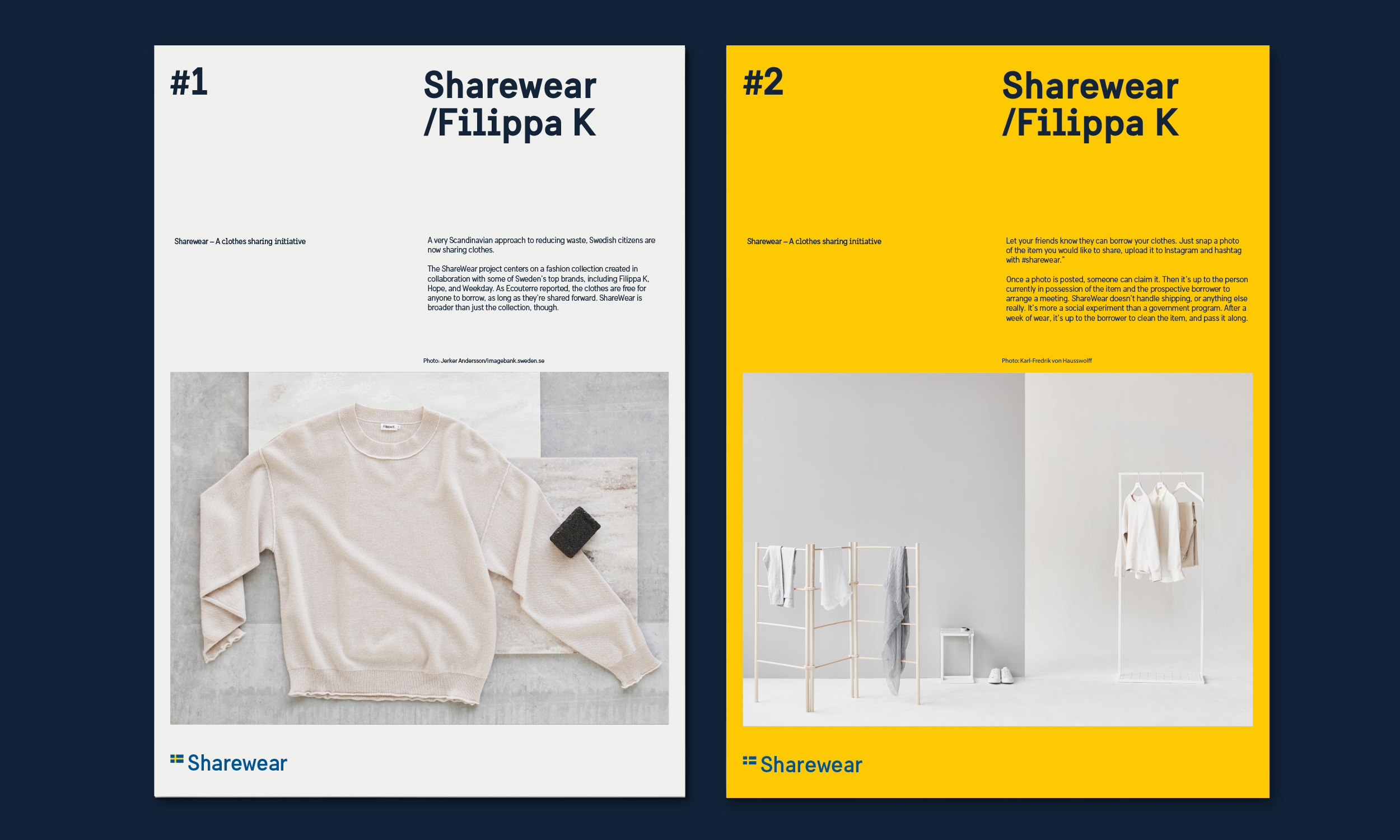The image is a rectangular composition featuring two separate flyers against a solid blue background. Each flyer occupies half the image, with the left flyer being white and the right one orange. Both flyers prominently display a product photograph accompanied by multiple lines of black text. The left flyer, titled "Number One: ShareWear / Filippa K," introduces ShareWear, a Scandinavian initiative focused on reducing waste by encouraging Swedish citizens to share clothes. It features a white long-sleeved shirt as the central image and provides details about the collaboration with top Swedish brands like Filippa K, Hope, and Weekday. According to Ecoture, the clothes are available for free borrowing as long as they are shared forward.

The right flyer, labeled "Number Two," continues the ShareWear narrative, explaining the process of lending clothes through social media. It instructs users to photograph the item they wish to share, upload it to Instagram with the hashtag #ShareWear, and arrange a meeting with interested borrowers. This flyer features an image of a wooden clothing rack, resembling three ladders, adorned with white shirts and other pieces of clothing. The ShareWear initiative is described as more of a social experiment than a conventional program, relying on community participation rather than structured oversight. Both images collectively highlight the ShareWear initiative's innovative approach to sustainable fashion and communal resource sharing.